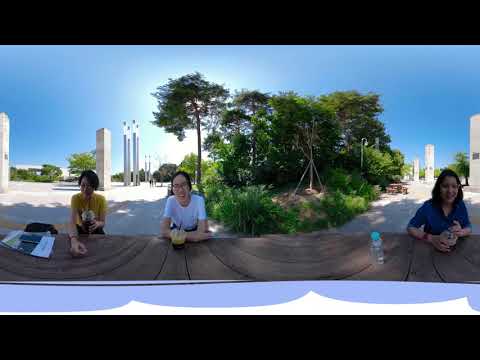In the image, three young Asian women are seated at a wooden picnic table outdoors, enjoying each other’s company. On the left, a woman with short dark hair is dressed in a yellow blouse, holding a drink in her left hand while her right hand rests on the table. Papers are scattered to her left. The middle woman, wearing glasses and a white short-sleeved shirt, is smiling at the camera. In front of her is a brown drink in a clear plastic cup, and her arms are resting on the table. The woman on the right, with shoulder-length dark hair and glasses, is wearing a blue v-neck shirt and also holding a drink. A water bottle is placed on the table in front of her. The table itself is made of wooden slats that appear slightly curved. 

Behind the women, the bright blue sky frames a lush background of trees and greenery. The scene also features scattered tall, skinny metallic structures that resemble small monuments or sculptures, adding a unique architectural element to the natural setting. The ground appears sandy or beige. The setting suggests that they are in a park or a nature reserve, where tourists might frequent. The image is bordered by a black frame at the top and bottom.